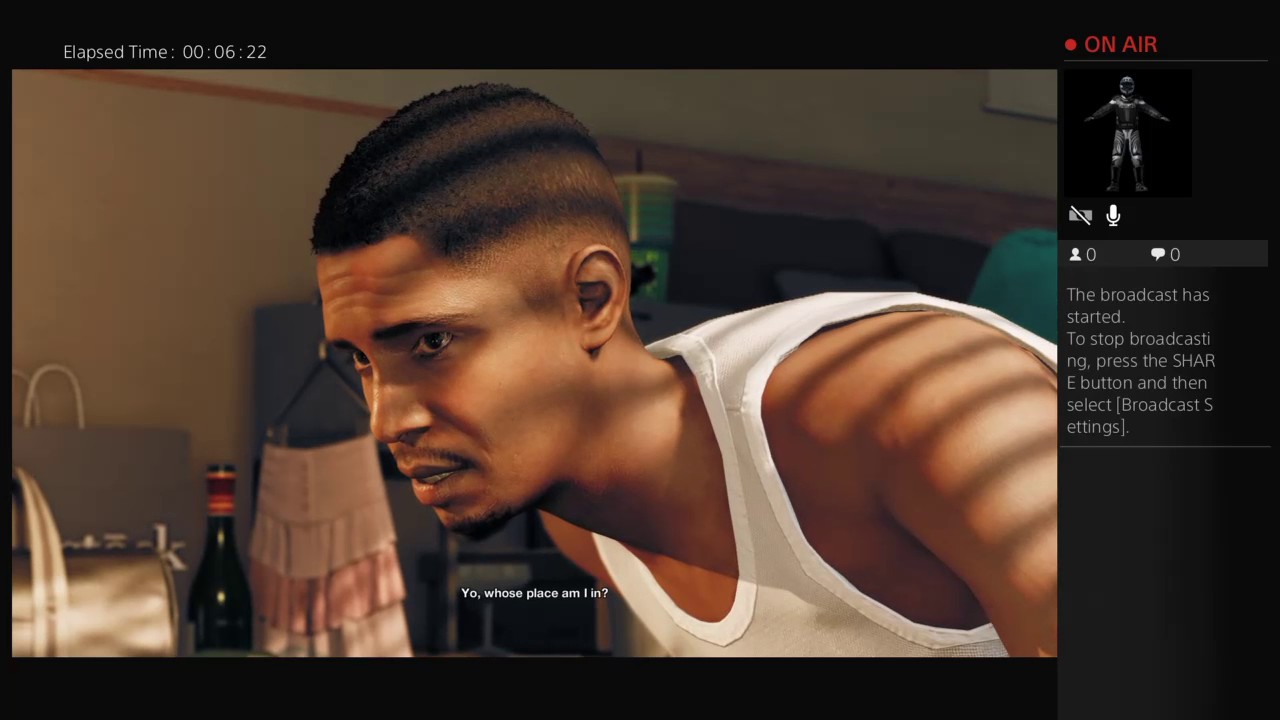A screenshot with a black background displays an elapsed time of 00:06:22. The screen prominently shows an "ON AIR" indicator in red, accompanied by a red circle. A man's profile picture is present, along with icons indicating zero by his profile picture and zero by the chat icon, suggesting no current viewers or messages. The broadcast is active, with text instructions advising that to stop broadcasting, one should press the "SHARE" button and then select the broadcast settings (noted in brackets).

The image features a man wearing a white T-shirt, with shaved hair, brown eyes, a faint mustache, and a more pronounced goatee. The background includes various items such as a bottle, a shopping bag, and a skirt hanging up. The walls of the room are brown. Below the man, white text asks, "Yo, whose place am I in?"